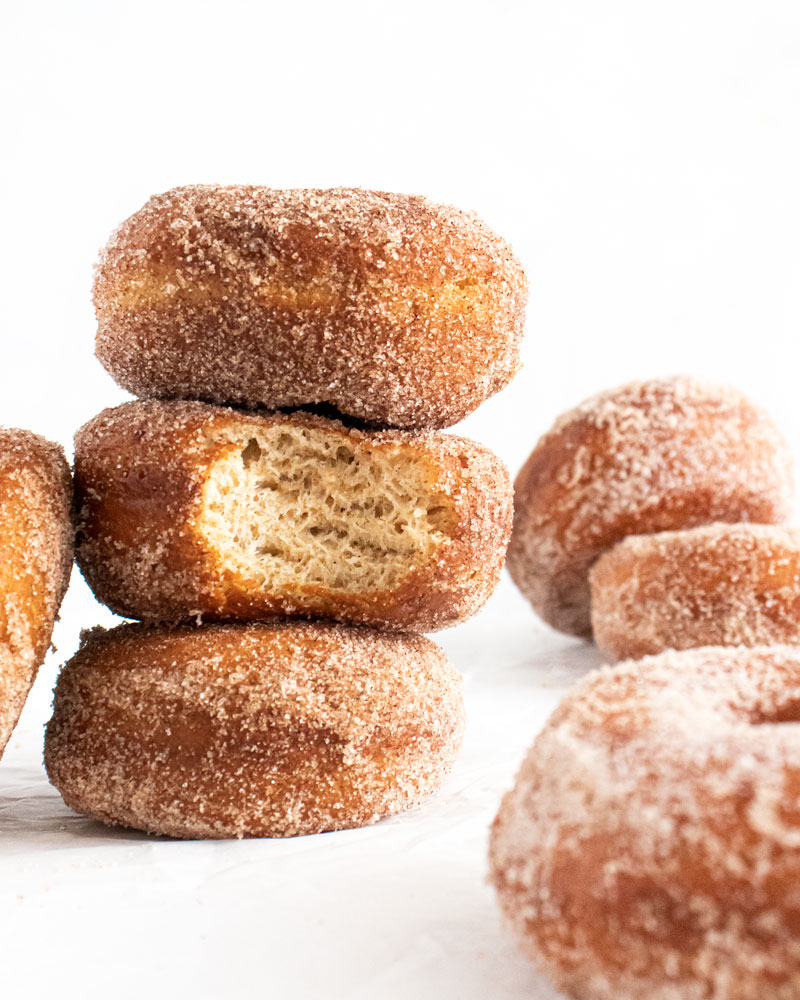The image is a professionally taken, close-up photograph of cinnamon sugar-covered doughnut holes arranged on a white background with expert studio lighting. At the center of the image, three doughnut holes are meticulously stacked on top of one another, creating the focal point of the composition. The middle doughnut hole has a noticeable bite taken out of it, revealing its soft, delectable interior. Surrounding this central stack, there are various other doughnut holes positioned in a scattered manner, creating a balanced visual arrangement. On the left-hand side, one doughnut hole leans against the central stack, partially coming into the frame. Additional doughnut holes can be seen on the right-hand side and the upper left, though they are intentionally blurred to keep the focus on the central stack. The clarity of the image is so high that individual sugar crystals and cinnamon specks on the doughnut holes are distinctly visible, enhancing their mouth-watering appeal. This image appears to be crafted for an advertisement, showcasing the sugary, fried dough treats in an enticing manner.